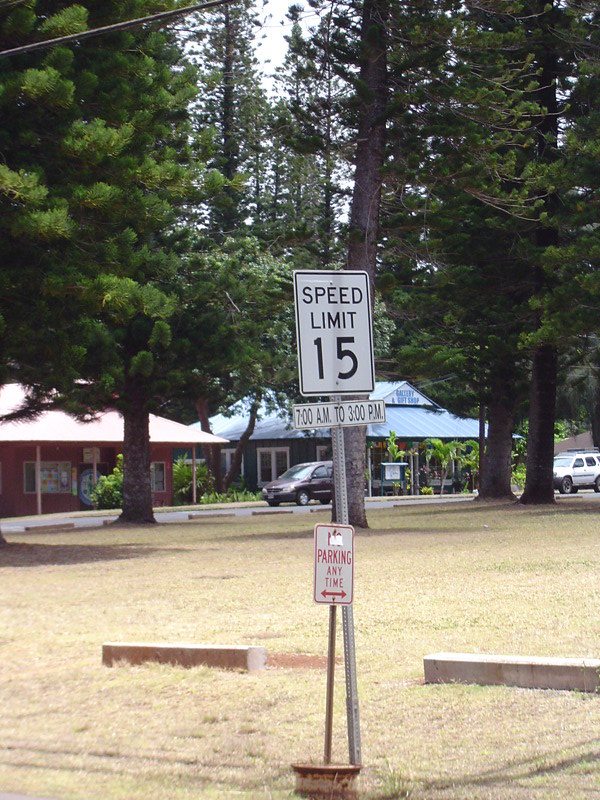This is a detailed color photograph in portrait orientation, capturing a small park or potential school zone. The central focus of the image is a prominent speed limit sign that is a white vertical rectangle with bold black text reading "Speed Limit 15" in large font. Below it, a horizontal panel specifies the time frame, "7 a.m. to 3 p.m." This sign is affixed to a tall steel post. Positioned in front of this is another, shorter sign, a white vertical panel with red lettering that states "No Parking Any Time," accompanied by a red arrow pointing left and right.

In the background, there's a gravel lot equipped with a couple of concrete stops. Beyond this lot lies a mix of residential and commercial areas. Two businesses, set back in the photograph, are partially obscured by landscaping, which includes small palm trees. Additionally, you can spot a bulletin board filled with numerous postings, suggesting the possible presence of a school or an active business. Tall pine trees frame the backdrop, with several parked cars and others traveling just visible through the tree line. The composition of the image is in a photographic representationalist realism style.